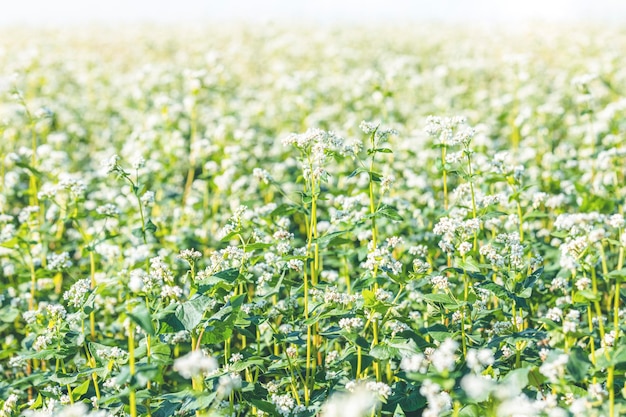The landscape-format photograph captures an expansive field of delicate plants, each standing a few feet tall. These plants exhibit bright chartreuse neon green stems and slightly darker green leaves. Topping each stem are clusters of small, white flowers that create a soft, ethereal effect. In the forefront, the closest stems and flowers are artistically blurred, drawing the eye to the sharply focused flowers just behind them. As the field stretches out, the flowers gradually fade into indistinguishable dots, giving the impression that the field extends for miles. The image is bathed in bright morning light, and the distant background appears slightly foggy, contributing to the dreamy quality of the scene. The repetitive elements of vibrant green stems and countless tiny white flowers fill the entire image, maintaining a consistent visual theme throughout.